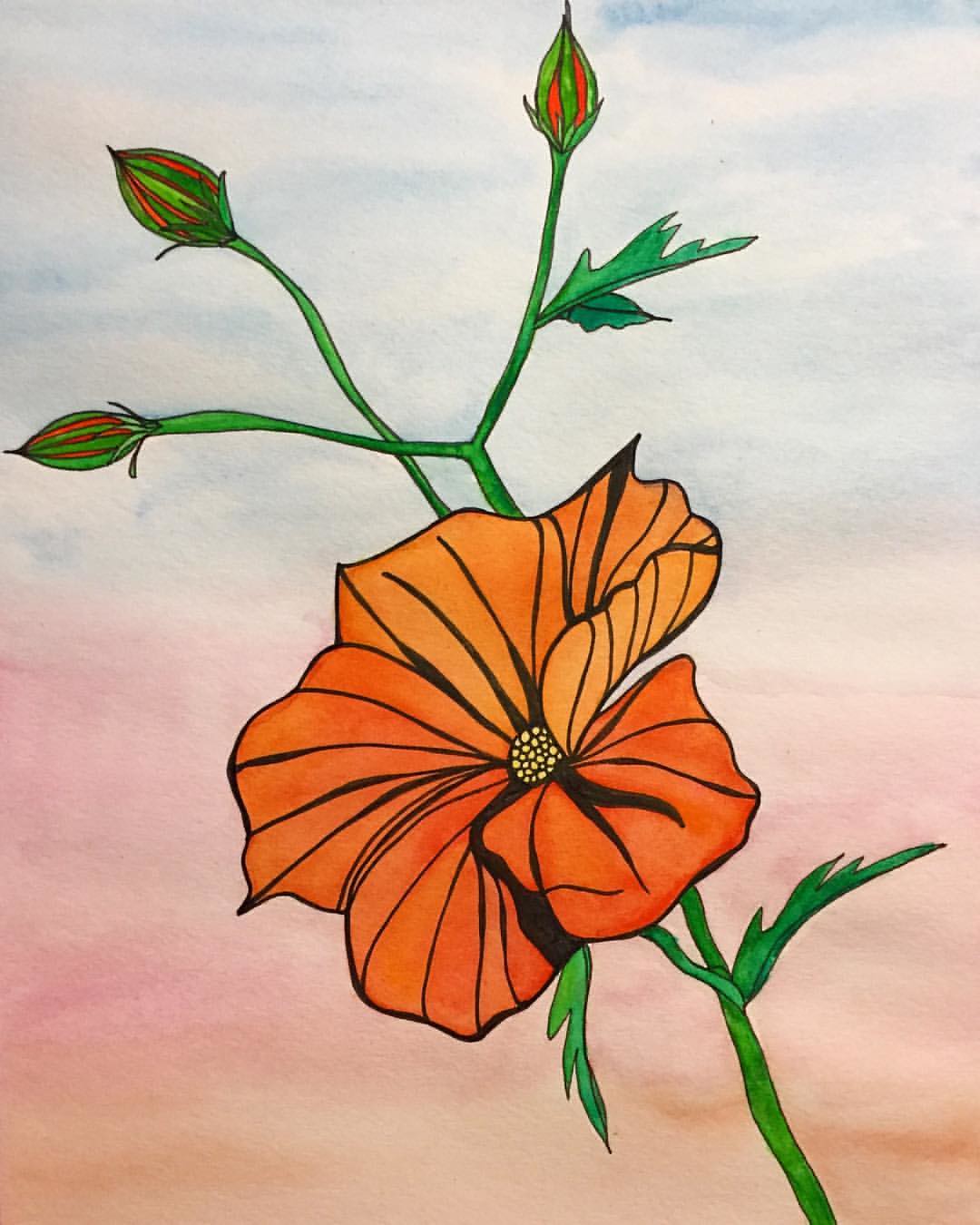This colorful, portrait-format illustration masterfully blends colored pencil and marker with watercolor, showcasing a strikingly attractive orange flower. The flower is outlined in black, which also accentuates the contours of its large, vibrant petals. At the center of the flower is a small yellow dot, adding a touch of brightness. The substantial green stem, which emerges diagonally from the bottom right to the top left of the image, supports the main blossom and branches off into three additional buds, hinting at future blooms. Each bud is tinged with lines of orange, suggesting the color they will eventually unfurl. Accompanying the flowers are a few small green leaves, adding to the natural motif. The background transitions beautifully from a blue, cloud-like sky at the top to a pinkish hue below, evoking the dreamy essence of a sunset or sunrise. This creates a visually appealing contrast to the rich colors of the flower and its foliage.